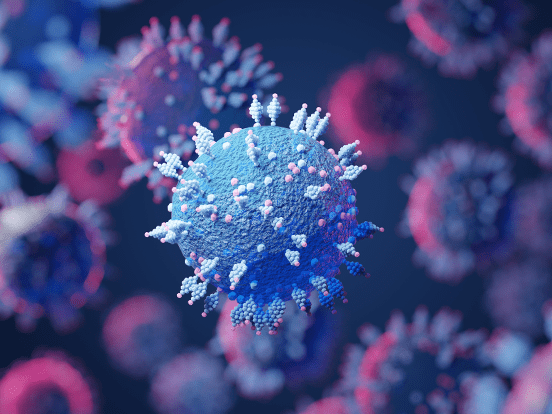This color image is a detailed computer-generated rendering of what appears to be a virus or molecule, reminiscent of a coronavirus. Dominating the center is a blue orb with a textured surface, speckled with white and pink spots. Short, stubby stems or spikes extend from various points on the orb, which are primarily blue with pink tips. The foreground focuses sharply on this central orb, highlighting its intricate details and giving it a three-dimensional appearance. Surrounding the central figure, the background reveals a half dozen or so similar orbs, blurred and out of focus, in hues of pink and purple. These background orbs add depth to the image while maintaining a clear emphasis on the central blue structure. The overall color palette of the image includes various shades of blue, pink, purple, and fuchsia, creating a vibrant and somewhat surreal representation of microscopic life. The image is rectangular in shape, further framing this captivating central orb and its surroundings.